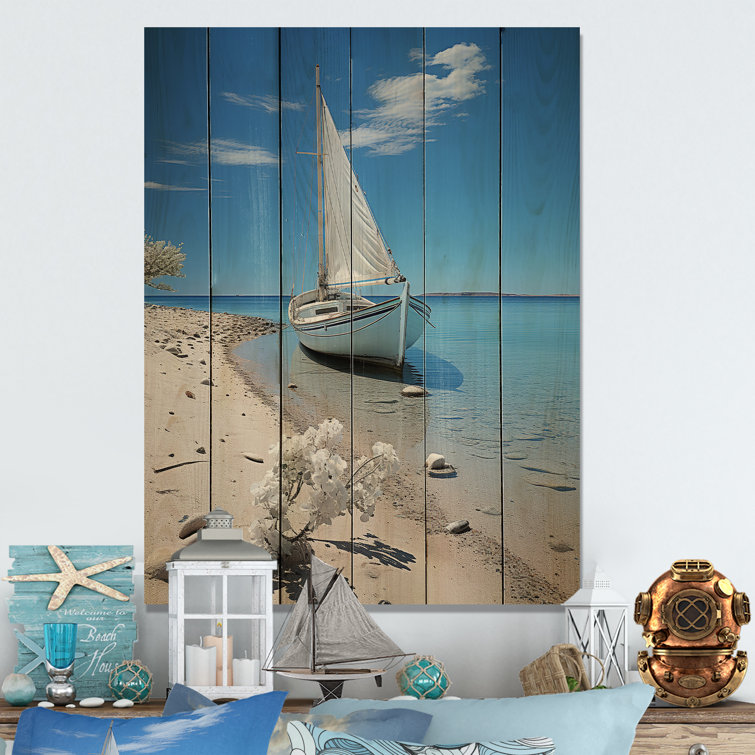A detailed painting of a tranquil seaside scene covers a section of a gray back wall, with the wood slats of the painting creating a textured background. The artwork features a pristine white sailboat with two windows and a drooping rope on either side, moored near a rocky sand-covered beach. An unusual blossoming tree emerges from the shore, adding a touch of whimsy. Above, a bright blue sky is dotted with a few wispy white clouds, enhancing the serene atmosphere.

On a shelf beneath the painting, a variety of nautical-themed objects are symmetrically arranged. Starting from the left, there is a picture of a starfish with the words "Welcome to our beach house" against a light blue background. White stones are scattered in front of it, adding a touch of nature. A white wooden lantern with three candles, two white and one tan (with the tan one in the middle, lit), stands nearby. Next to this, a model sailboat with three sails complements the coastal theme.

Adjacent to the sailboat, a green orb encased in macrame rope rests beside a tipped-over wicker basket, with green contents spilling out. Another white lantern, this one empty, adds to the display. In the right-hand corner, an antique brass scuba diving helmet, reminiscent of 1940s designs, provides a vintage maritime touch.

On the far-right side, a blue pillow featuring the same sailboat depicted in the painting ties the theme together, while a blue glass cup with a silver chrome handle adds a final charming detail to the beach-inspired decor.